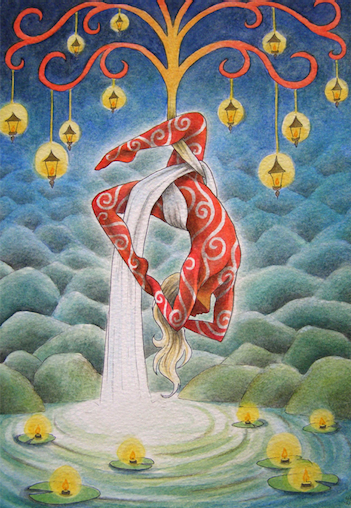The image depicts a striking scene of a performer, elegantly suspended upside down from a white silk that transforms into an intricate, tree-like chandelier at the top. This chandelier-like structure, which blends shades of orange and red, extends branches that curl and hold numerous lanterns with glowing flames.

The performer, a woman in a vivid red bodysuit adorned with intricate white swirls, gracefully arches her back, extending her torso downwards and reaching back to grasp her right leg with both hands. Her long, blonde hair flows downward, adding to the fluidity of her pose. The white silk she is suspended from wraps around her body, threading between her legs and securing her in this elegant position.

Beneath her, the silk appears to cascade like a waterfall into a serene pool of water, disrupting its surface into gentle ripples. In the water below, seven lily pads float, each illuminated by a small tea light, casting a warm, flickering glow. The background features grayish-green rocks that fade into a dark blue, creating a dreamy, ethereal atmosphere for this captivating acrobatic display.